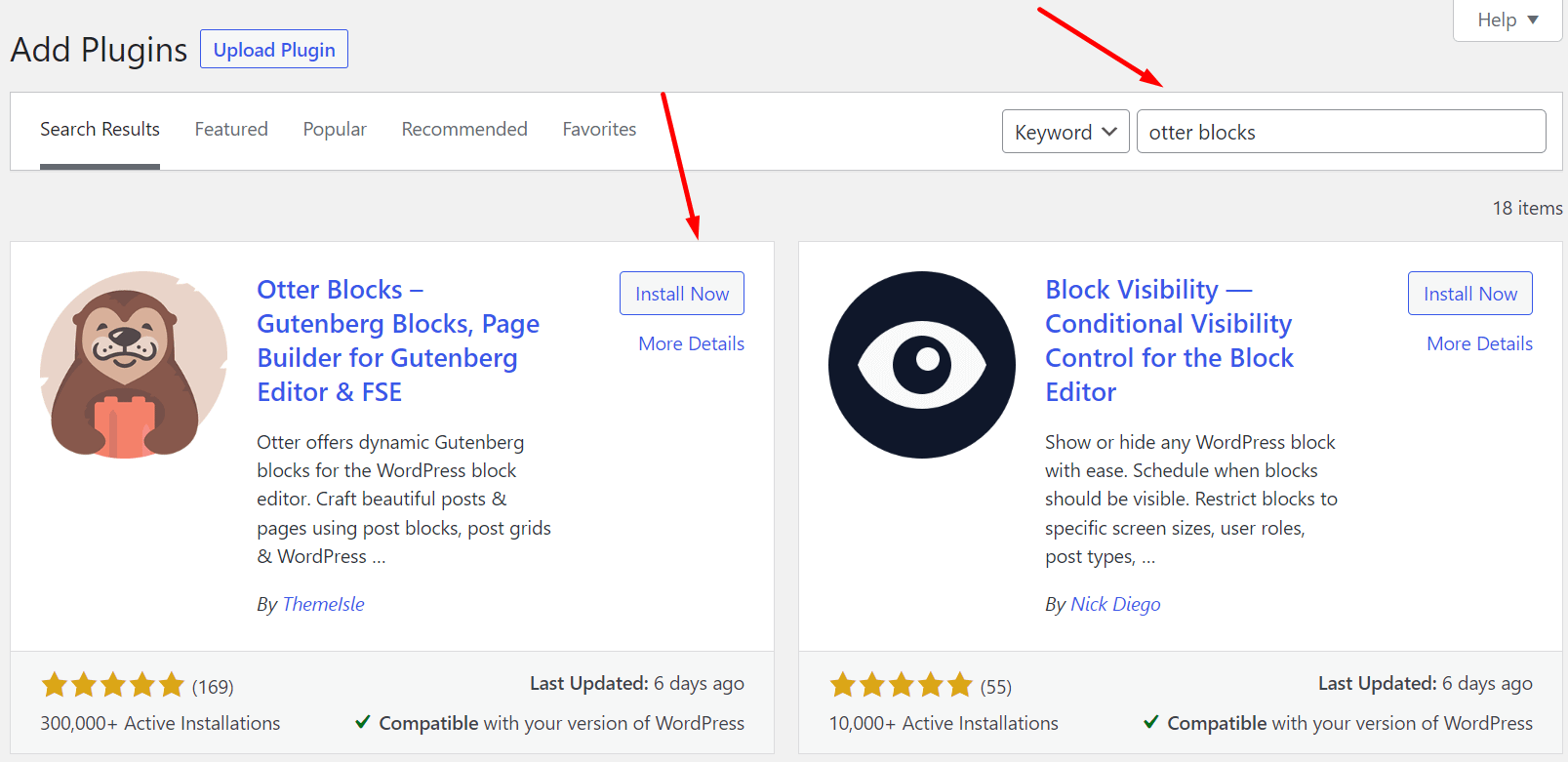The image showcases a user interface for adding a plugin in a WordPress environment. At the top, there's a gray-bordered header featuring the text "Add Plug-in" in black. Adjacent to this, a rectangular box with a blue border reads "Upload Plug-in." Beneath this, there's a white section labeled with several clickable categories, including "Search Results," "Featured," "Popular," "Recommended," and "Favorites."

A dropdown menu labeled "Keyword" is positioned above a search box titled "Other Blocks," which features a red arrow pointing towards it for emphasis. Below this search box, to the right, there is another white box displaying an image of a brown teddy bear on the left side. Next to the bear, in blue text, it reads "Otter Blocks - Gutenberg Blocks Page Builder for Gutenberg Editor and FSE." This section includes an "Install Now" button with a red arrow pointing at it.

At the bottom of the description, the text elaborates on the plugin's features, stating: "Otter offers dynamic Gutenberg blocks for the WordPress block editor. Craft beautiful posts and pages using post blocks, post grids, and WordPress." The plugin has a five-star rating displayed prominently.